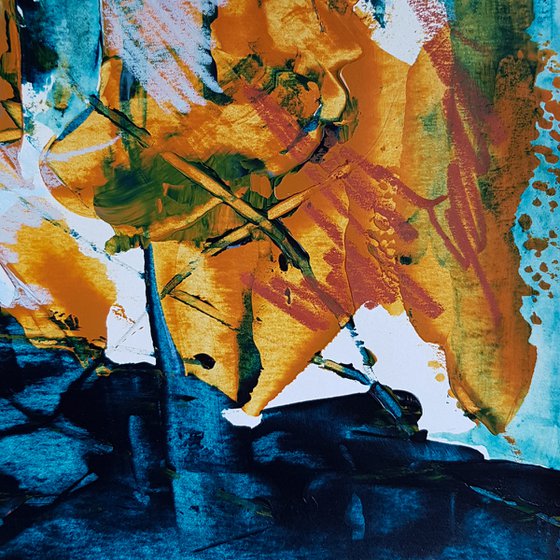This image showcases an abstract painting characterized by a mesmerizing interplay of colors and shapes that evoke various imaginative interpretations. Dominating the bottom section are intricate mixes of light blue and dark blue hues, which blend seamlessly to create a dynamic background that stretches from the left corner to the right corner. Throughout this expanse, patches of navy blue emerge, interspaced with regions of lighter blue. Above this, on the right side, a wash of light aqua appears, adorned with small brown and red dots.

Central to the composition is an intriguing amalgamation of gold, orange, yellow, and green paints forming a striking focal point. This section, resembling a five-pointed star with three points on top and two on the bottom, is further accentuated by green splatters within the gold paint. Additionally, there are red lines coursing through this vibrant area, complemented by blobs of yellow and streaks of green, reminiscent of finger painting techniques.

Amidst these colors, the painting evokes the visual of a scene akin to an animal with a bridle, featuring a white nose and a yellow and blue ear. A sense of presence is suggested with outlines that might represent a sleeve and hand, though these details are subject to the abstract nature of the art. This impression integrates with surrounding elements such as a blue cliff-like formation and subtle white cloud-like wisps in the background, creating a multifaceted and immersive visual experience.